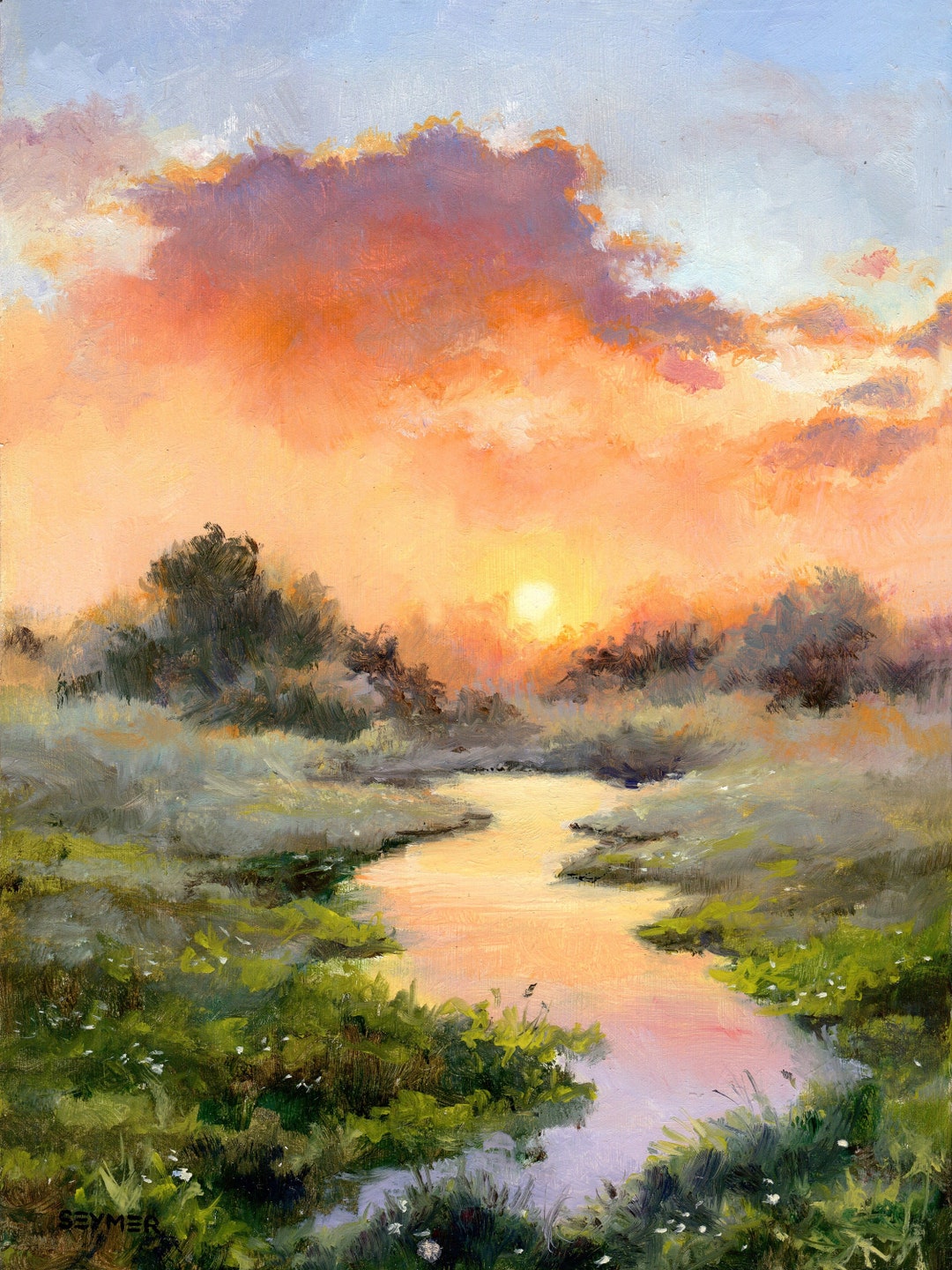This painting depicts a serene outdoor landscape, characterized by a zigzagging stream or brook that winds through a lush meadow. The stream starts narrow in the foreground, expanding as it flows deeper into the scene. The banks are decorated with rich green grass, low shrubs, and sporadic patches of white flowers blooming both in the foreground and mid-ground.

In the distance, the scene transitions into a fog-covered area with silhouetted trees, hinting at an early morning or late evening setting. Above the treeline, the sky is ablaze with the colors of a sunrise or sunset, featuring a balance of blue and white at the top, transitioning into orange, red, and purple hues closer to the horizon. The sun sits centrally in the sky, casting its warm light across the landscape and reflecting in the stream below, which mirrors the vibrant colors of the sky. Wispy clouds, tinged with purple and yellow, add texture to the sky, enhancing the overall ethereal quality of the scene.

This masterful oil painting, with its detailed brushstrokes, captures the tranquil beauty and subtle shifts in light and color, creating a picturesque and harmonious depiction of nature.